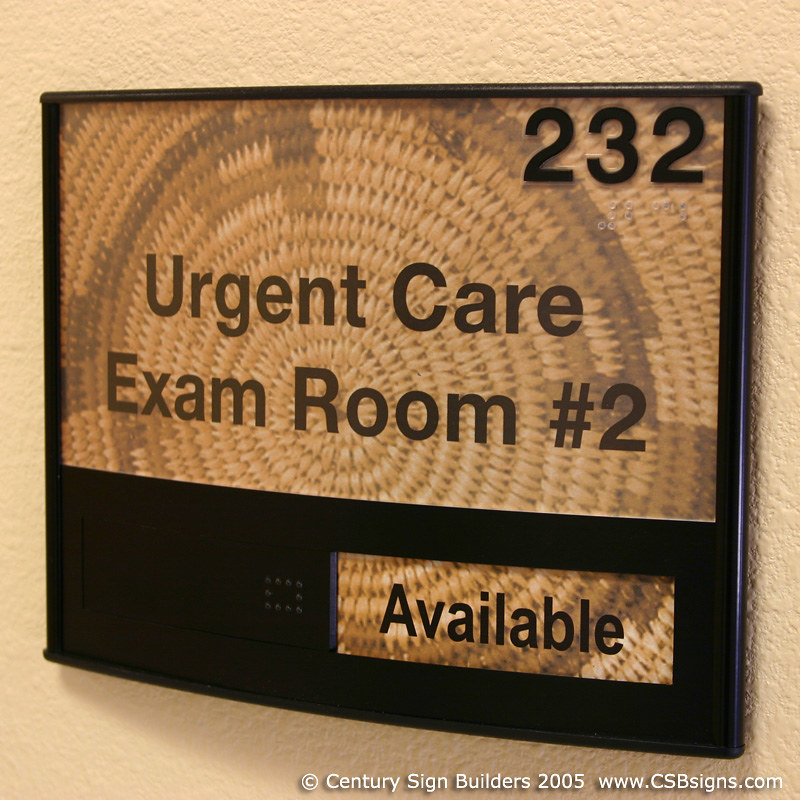The image depicts a room number sign mounted on a textured wall of a creole magnolia color. The sign features a black plastic frame with a transparent upper section that reveals a background resembling a woven basket pattern with dark brown or black concentric circles. The sign includes several key elements: at the top left corner, the room number "232" is displayed in black text; beneath it, in the middle section, the text reads "Urgent Care Exam Room Number 2." In the bottom left corner, there is a sliding piece of black plastic that indicates the room's status, currently showing "Available." A small square in the bottom right contains a white “C” in a circle, followed by the text "Century Sign Builders 2005, www.csbsigns.com,” also in white. The plastic frame covering the sign has a textured background visible through the transparent upper portion, blending modern signage with a classic woven aesthetic.